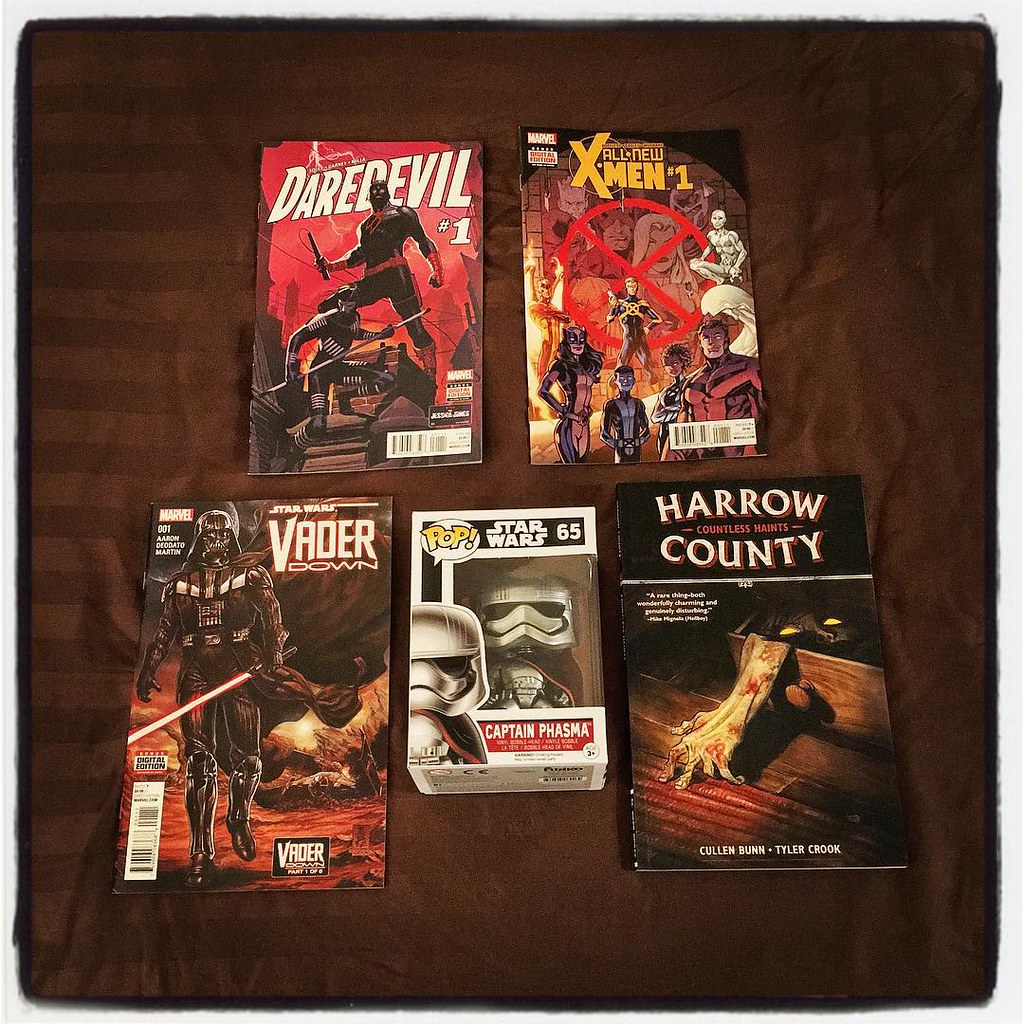The image depicts a collection of five items placed on a surface covered with brown fabric featuring horizontal dark and light brown stripes. At the top left is a comic book titled "Daredevil No. 1," showcasing a black, white, and red cover with two characters engaged in combat. To its right is another comic book, "All New X-Men No. 1," with the title in bold yellow font at the top, a red circle with an X, and several superheroes, including a character with blue skin and another with a feline mask. Below these, on the bottom left, is a comic book titled "Star Wars: Vader Down," displaying Darth Vader in his iconic black costume and helmet, wielding a red lightsaber against a red background. In the center of the image is a Funko Pop figurine in a white box, labeled "Pop Star Wars 65 Captain Phasma," the figure depicting Phasma in silver armor. To the right of the figurine is a book, "Harrow County: Countless Haints" by Cullen Bunn and Tyler Crook. The book has a black cover featuring a drawer with yellow eyes peeking out and a bloodied arm. The setting appears to be indoors, lit by warm lighting.